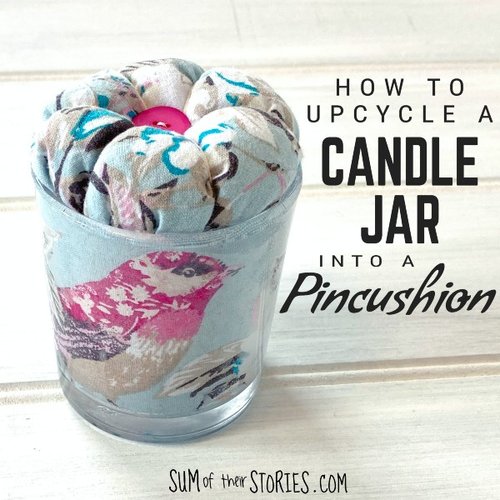This image is a photograph of a craft project showcasing how to upcycle a candle jar into a pincushion. The main element is a clear glass jar, formerly a candle holder, that has been transformed. The jar features a decorative pattern of a bird with a pink head and brown body, surrounded by small floral designs, which appears to be decoupaged or possibly a fabric placed inside the jar. The pincushion's top is adorned with multiple sections of colorful fabric, predominantly light blue with dark blue, white, and pink shapes, cinched with string or thread to form small bulging sections, topped with a prominent pink button at the center.

The entire setup rests on a white wooden surface. In black lettering on a white background to the right of the jar are the words, "how to upcycle a candle jar into a pincushion," with "candle jar" in larger letters and "pincushion" in a distinct font. At the bottom, the text reads, "someoftheirstories.com."